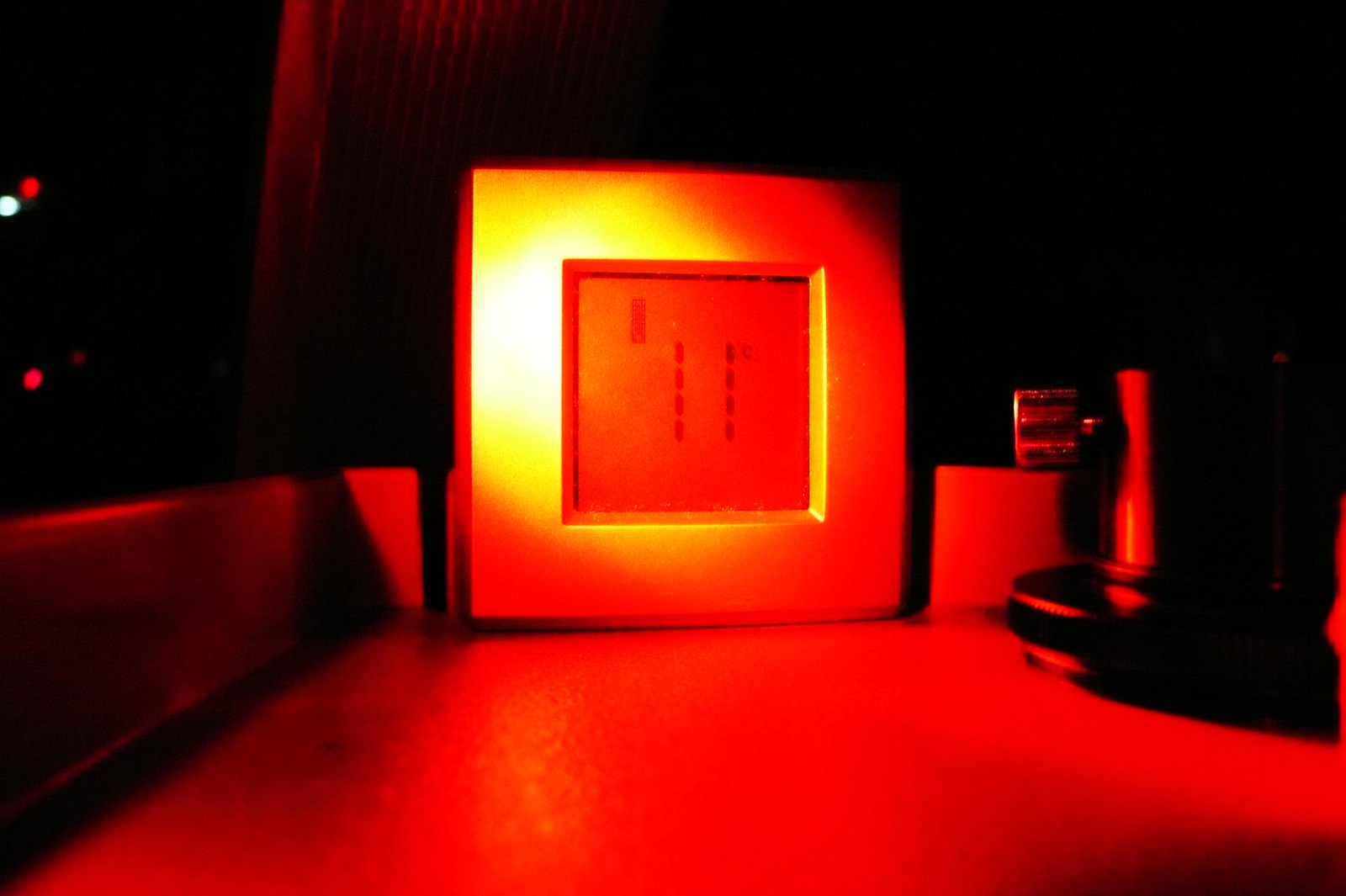The photograph captures a scene illuminated predominantly by red light, which casts an intense, almost surreal orange hue over everything, especially the orangey-brown countertop where the focal object rests. The object is a square, featuring a silvery metal-colored frame, although the red light distorts its true color. At the center of this framed display, there is a black LCD screen showing the number "11" with a small "C" positioned to the upper right. To the left of the "11," there appear to be oriental letters or markings. The background is mostly dark with indistinguishable objects, though faint vertical lines and a couple of faint red and white dots are faintly visible to the left. To the right of the square object, there are shadowy, unidentifiable items. The photograph's curious lighting and composition lend it a mysterious and intriguing atmosphere.